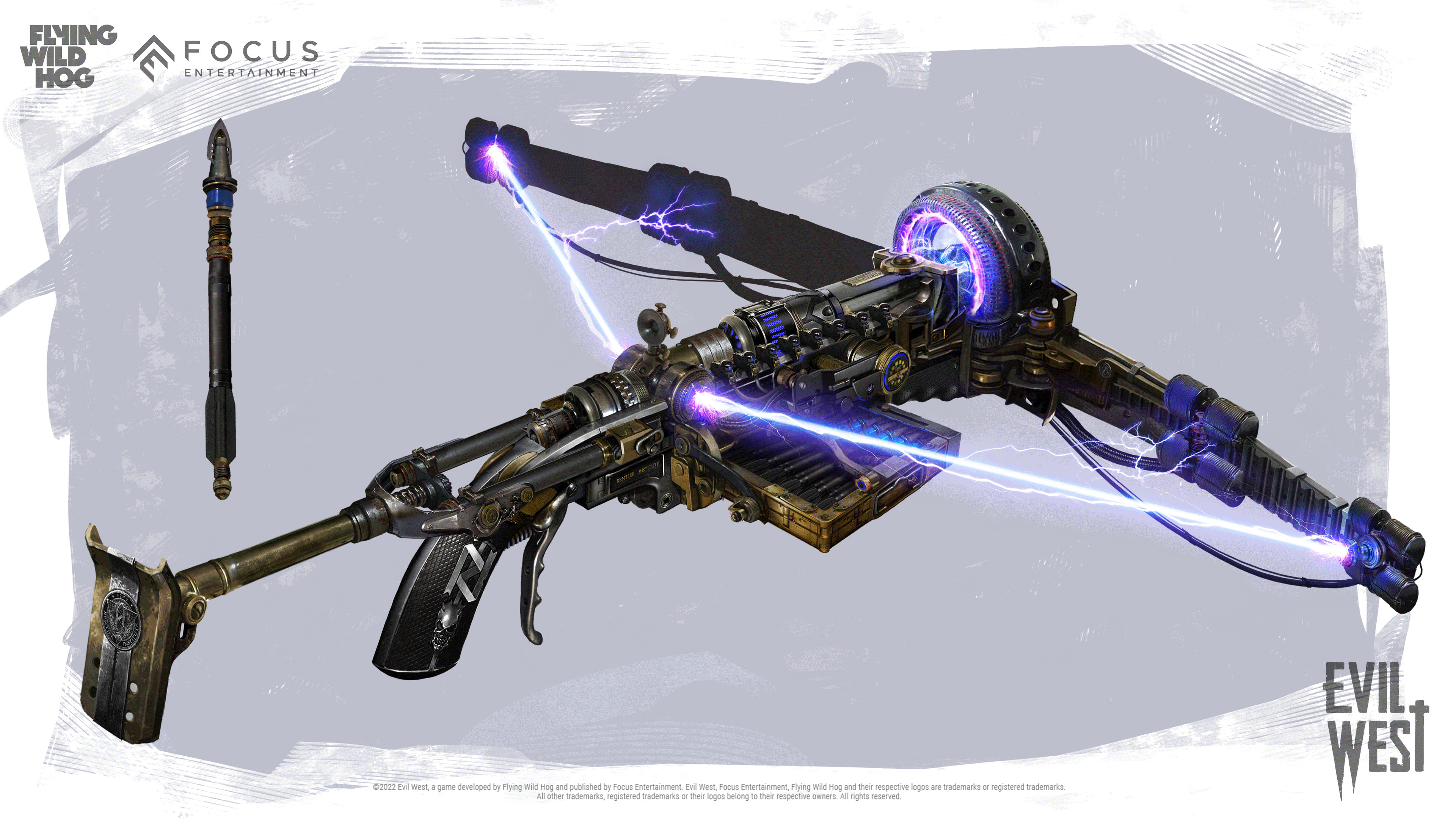The image appears to be a highly detailed, futuristic weapon resembling a crossbow or gun, predominantly black with intricate gray stripes and laser-like graphics. On the left side, there is a distinct shoulder rest, followed by a short barrel and a main handle with a trigger handle positioned behind it. Midway along the weapon, a cartridge is visible on the right side, presumably for ammunition. Extending towards the front, a long crossbar structure mimics a crossbow setup, and a small tire-like component with lightning designs is situated at the center front. Purple light accents appear to highlight its high-tech nature. The background of the image features a light purplish-gray gradient, providing contrast to the weapon. The image includes text with "Evil West" in gray letters at the bottom right, while the top left corner showcases "Flying Wild Hog" and "Focus Entertainment" in similar gray lettering. Overall, it conveys a sense of advanced, futuristic weaponry possibly from a video game context.